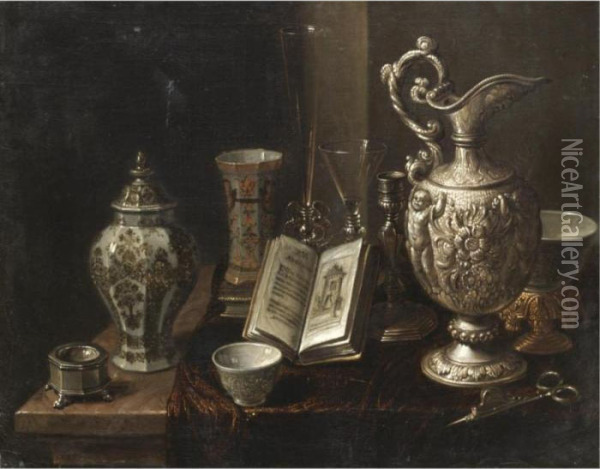The image depicts a realistic still life painting set in a dimly lit room, showcasing a variety of old-fashioned, ornate kitchenware. Arranged on a table covered with a goldish-brown tablecloth adorned with intricate patterns, you find an ensemble of finely detailed objects, including an urn on the left and a water jug with elaborate engravings on the right. Scattered amongst them are various smaller vessels—a white porcelain cup, several mugs, a martini glass-like item, and other intriguing containers. There's also a candle holder and a bowl in the scene. Notably, an open book with partially discernible words and an illustration of a house lies in the middle. Adding a touch of modernity to this antique tableau is the text "NiceArtGallery.com" visible on the side. The overall somber lighting subtly highlights the shiny, silvery, and porcelain surfaces, emphasizing the craftsmanship and giving an impression of expensive, treasured heirlooms.